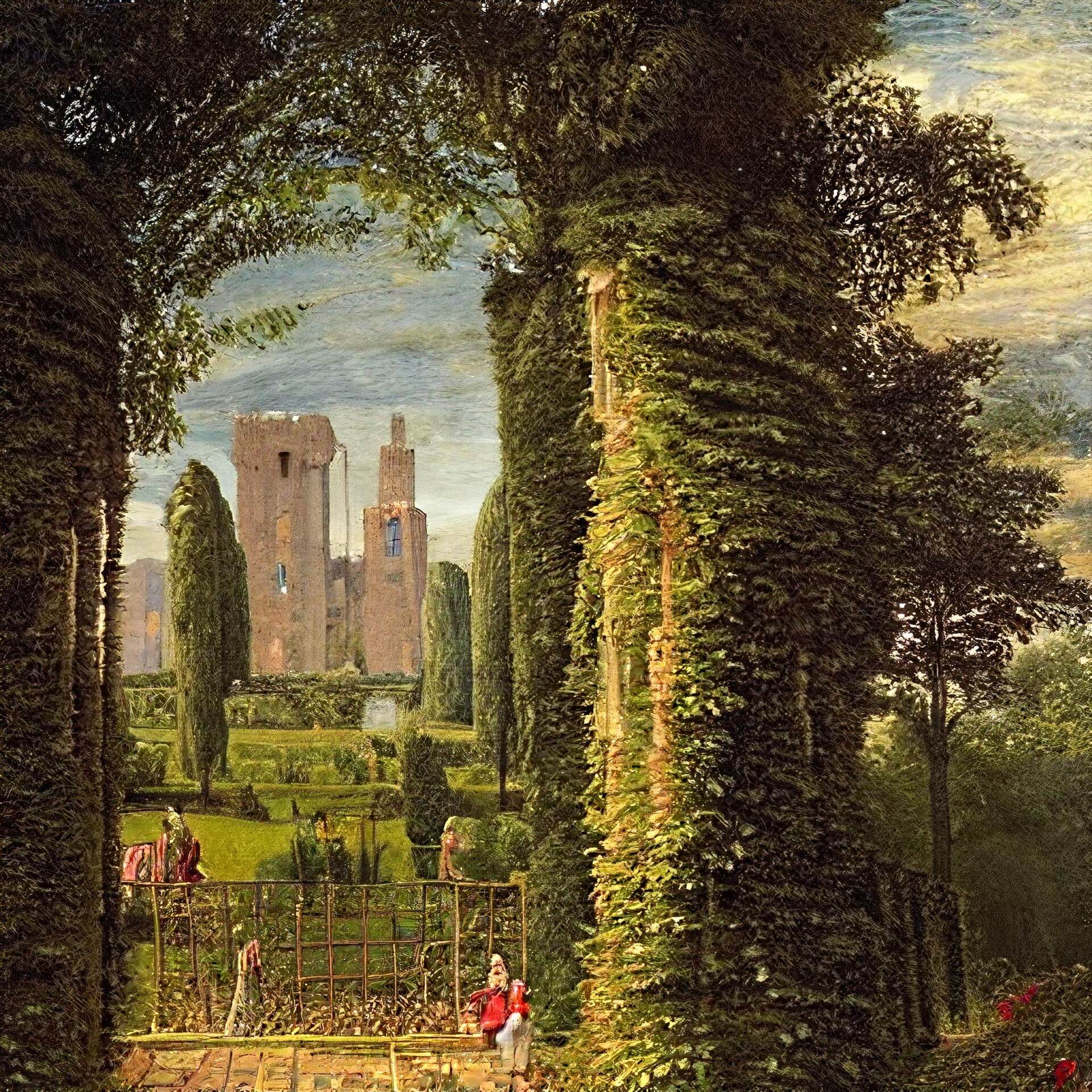The artwork depicts a verdant garden scene, dominated by an impressive lineup of tall, well-groomed trees. The focal point is a tall archway on the left side of the mid-ground, almost completely overgrown with vibrant green vines, barely revealing the pillars beneath. Through this archway, a path leads into the garden where a low fence stands before the trees. Among the foliage, the specific arborvitae trees are most prominent, characterized by their deep green color with patches of light green, possibly reflecting the sunlight. In the background, two tall beige buildings with sparse blue windows rise above the treeline, with the left building resembling a rectangular box with two upper-middle windows. A person in a red outfit, likely a dress, sits on a bench, adding a human element to the serene scene. The sky is a limited, bluish-green swath peeking through the dense canopy, shifting the visual focus to the lush vegetation and the architectural elements interspersed within it.